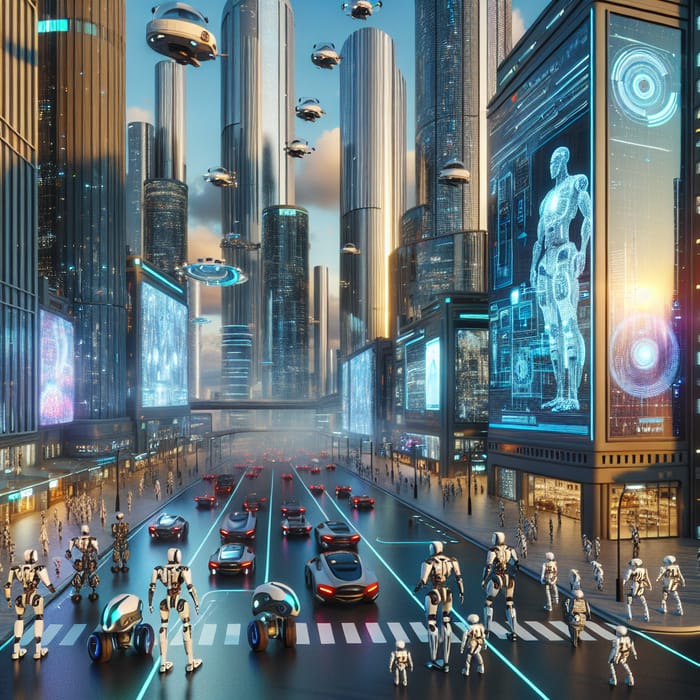The image is a detailed animated drawing or painting of a highly futuristic, sci-fi city street bustling with technology. Dominating the scene are various robots, both tall and short, predominantly colored in white and black, positioned all along a smooth, shiny black road marked with white stripes. Futuristic cars share the street with these robots, many of which give the impression of being children-sized beside their taller counterparts. Both sides of the street are lined with imposing, circular high-rise buildings featuring large digital billboards in shades of blue and black that display and explain robotic features. The muted color palette of the scene includes touches of reds and blues, adding to the high-tech ambiance. Above, the sky is filled with clouds and dotted with small UFO-like flying machines, resembling spaceships or drones, further emphasizing the advanced technological landscape. The overall scene captures a vivid interpretation of a future society deeply infused with robotics and advanced technology.